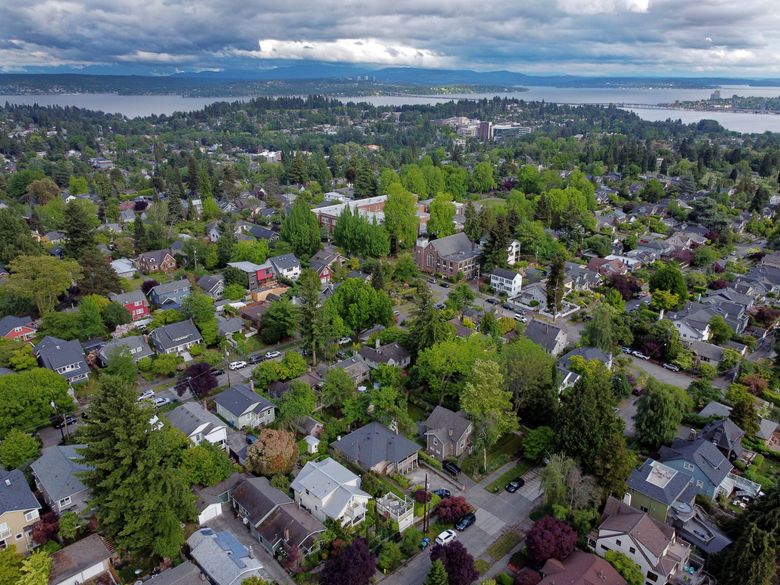This aerial photograph captures a sprawling suburban neighborhood filled with houses of varying architectural styles, predominantly two or three stories high with angled roofs. The homes are predominantly painted in shades of white, green, and tan, with many featuring grey or brownish-tan roofs. Interspersed among these homes are a few significant public buildings, including a large square institutional-style brick building, likely a school with a possible courtyard, an older two-story brick building with a gabled center and wings, and a white wooden-framed two-story building, possibly a church or town hall. The neighborhood is densely blanketed with tall, decades-old trees, both leafy and pine, contributing to a verdant canopy that covers much of the area. Streets crisscross the landscape, adding to the dense suburban layout. Towards the background of the image, a line of hills is visible, adorned with more trees and some buildings. Beyond the hills, a large body of water stretches out, with a bridge connecting an island-like landmass to the mainland. This scene is set against a backdrop of overcast sky with clouds extending to the horizon, adding a muted brightness to the daytime setting.